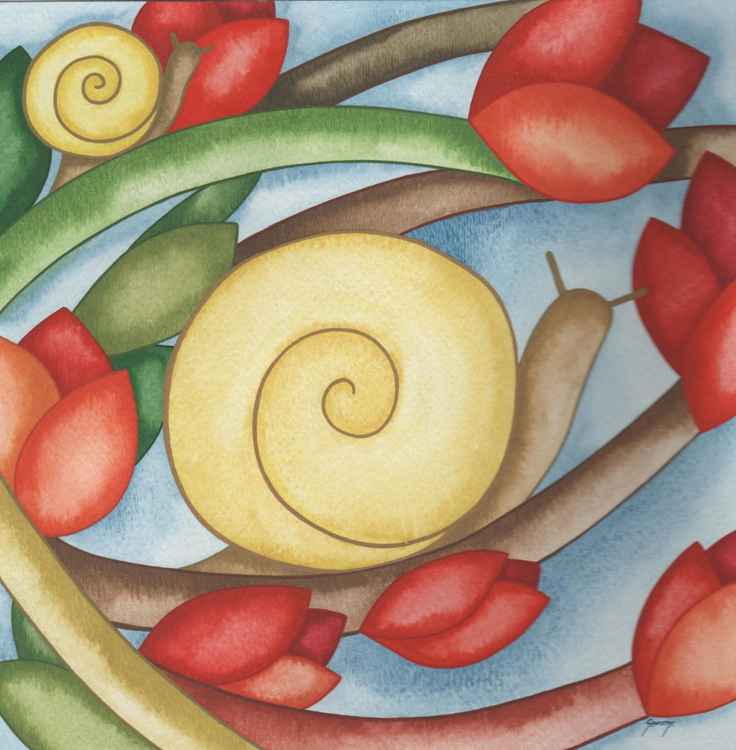This detailed handmade illustration depicts two snails amidst a vibrant floral scene. At the center, a large snail with a light yellow shell and a brown body is seen with its tentacles extended, crawling along the brown stem of a red tulip. Towards the upper left corner, there is a smaller snail of the same coloration, navigating a green stem of another red tulip. The background showcases a rich, blue hue that enhances the array of green leaves and red flowers, predominantly resembling tulips, with their stems varying in shades of green, red, and yellow. The art style suggests it could be created with colored pencils, given the visible shading, light reflections, and detailed textures. Though signed, the signature is too small to decipher. This evocative image captures the delicate interplay of nature, brought to life through meticulous handcrafted artistry.